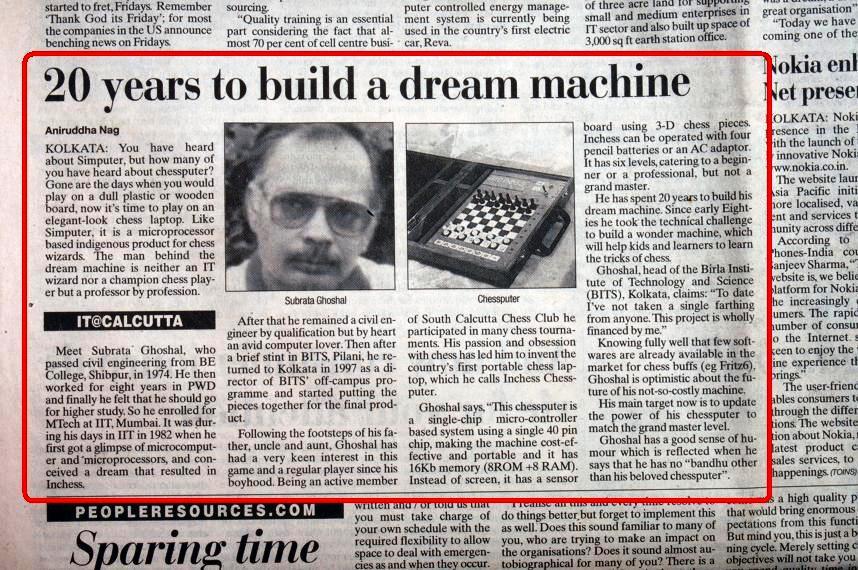This photo captures an old black-and-white newspaper clipping from Kolkata, distinguished by a red square border highlighting a key article titled "20 Years to Build a Dream Machine," authored by Anirudh Nag. The article narrates the advent of the innovative "Chessputer," a sophisticated, microprocessor-based chess device envisioned to replace traditional plastic or wooden boards. It introduces Subrata Ghoshal, the pioneering professor behind this ingenious product, portrayed in the included photograph. Ghoshal, described with thinning hair, aviator-style reading glasses, and a mustache, is pictured in the second and third columns, while the adjacent third column features an image of the Chessputer itself, resembling an electronic board game with black and white pieces. The article highlights the Chessputer as an elegant, laptop-like device poised to revolutionize the game for chess enthusiasts.